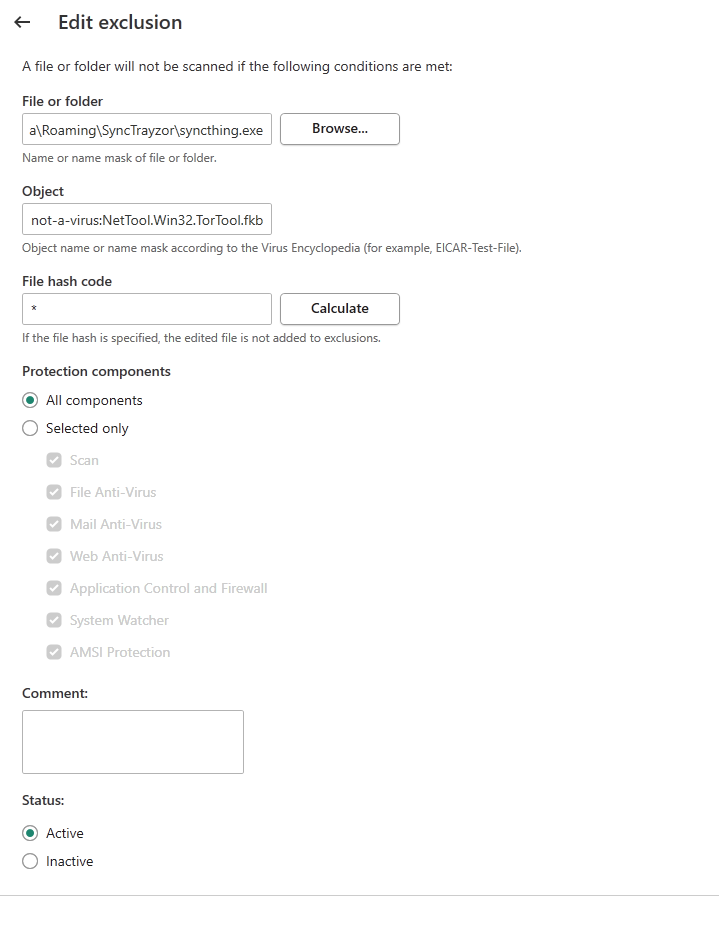The image features a detailed user interface for managing exclusion settings, displayed against a plain white background.

In the upper left-hand corner, there is a black arrow pointing left, accompanied by bold black text reading "Edit Exclusion". Below this is a line of regular-sized black text stating, "A file or folder will not be scanned if the following conditions are met."

Underneath this, the label "File or Folder" is displayed in bold text. Adjacent to this, there is a box containing the text "A slash roaming slash sync tracer slash sync thing dot exe." Next to the box, there is a rounded button outlined in black with bold text, "Browse…".

Following this section is some gray text that clarifies, "A name or name mask for a file or folder." Below this is another search bar labeled "Object" in black text, containing the value "Not-A-Virus, NetTool.Win32.TorTool.fkv." Further explanation in gray text follows, "Object name or name mask according to the virus encyclopedia (e.g., EICAR-test-file)."

Next is a section titled "File hash code" in bold black text, with an accompanying box containing a single black star. Adjacent to this box is a rounded button outlined in gray with the text "Calculate." Below lies a line of gray text, "If the file hash is specified, the edited file is not added to exclusions."

Further down is a header labeled "Protection components" in bold black text. Below this, there are two circular buttons: the first filled dark green, labeled "All components," and the second, an unselected white button with a gray outline, labeled "Selected only."

A list follows, each item marked by a black square with a white checkmark. The seven items include:
1. Scan
2. File Antivirus
3. Mail Antivirus
4. Web Antivirus
5. Application Control and Firewall
6. System Watcher
7. AMSI Protection

At the bottom, bold black text reads "Comment" above a gray-outlined white rectangle, and below this, another section titled "Status" in bold black text. Lastly, there are two buttons: one labeled "Active" filled in dark green, and another labeled "Inactive" with a white center and gray outline.